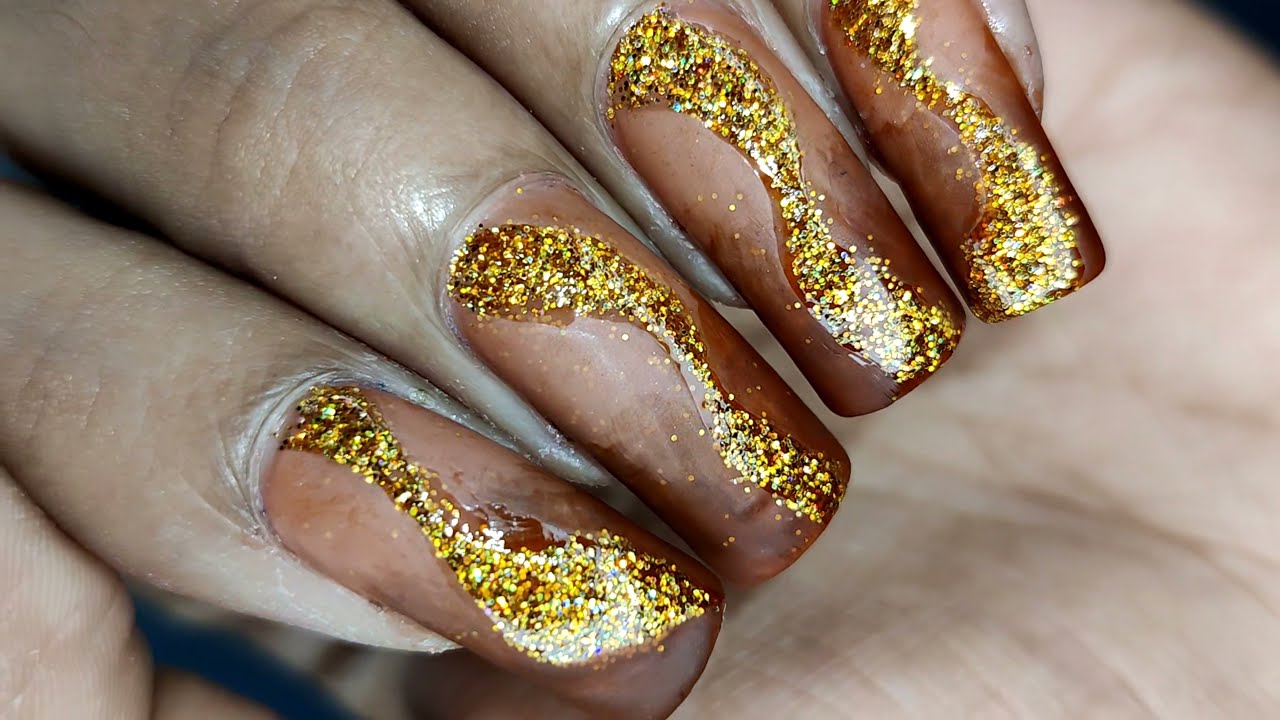This photograph is an extreme close-up of a person's left hand, highlighting their olive-skinned four fingers curled over their palm. The image is centered on the elaborate nail art adorning their long, fake nails. Each nail is painted in a tannish red hue and features intricate, gold glitter swirls that slither from the base to the tip. The glitter appears almost like glitter glue, adding a touch of sparkle to the nails. The background is a blurry view of the person's palm, filling the entire frame. The colors visible in the image include tan, brown, blue, gold, red, and white, creating a visually striking composition that resembles a photo from a nail art website.